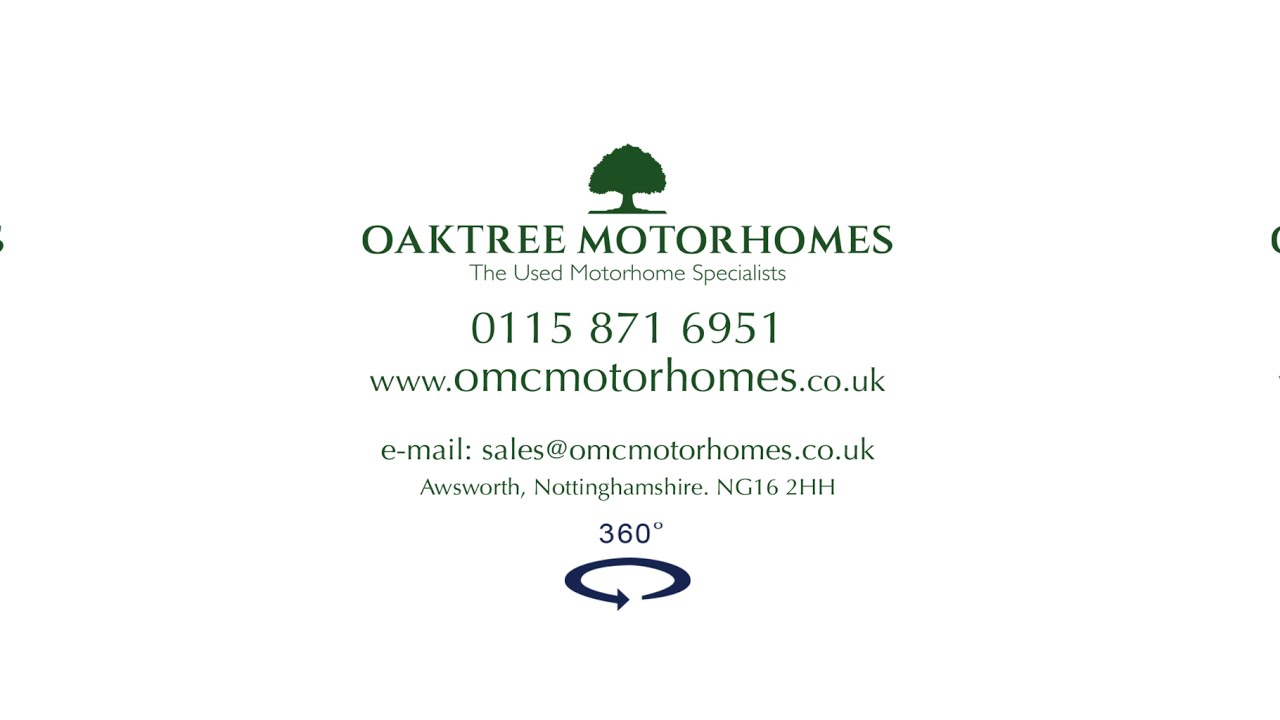The image features a business card-like advertisement with a white background, showcasing details in dark green text. At the very top and center of the card is a green silhouette of a tree. Below the tree, in bold green capital letters, is the business name "OAK TREE MOTORHOMES." Directly under that, in blue letters, it reads "The Used Motorhome Specialist." The next line lists a phone number: "0115-871-6951." Following the contact number, there is a website URL, "www.omcmotorhomes.co.uk." After a small space, the email is provided: "sales@omcmotorhomes.co.uk," formatted as "Email: sales@omcmotorhomes.co.uk." Beneath this, in smaller text, is the location: "Osworth, Nottinghamshire, NG16 2HH." At the bottom of the card, there is a 360-degree symbol with an arrow forming a circular shape around it.